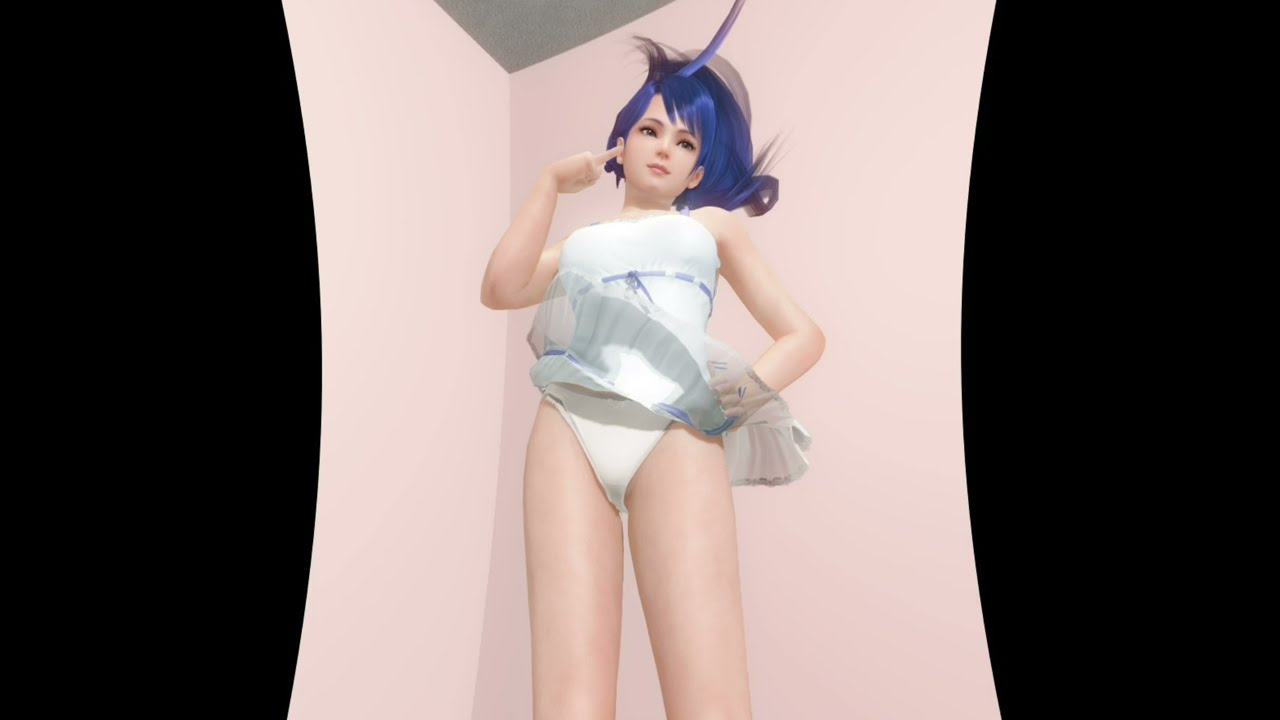The image is a detailed digital drawing of an anime-style young woman with fair skin and neon indigo blue hair, which is relatively straight. She dons a white dress with a lavender ribbon just under her chest, and the skirt of her dress is being blown upward, revealing her white bikini bottoms. The woman is positioned against a soft pink background, which shows a corner of a wall with black edges on the left and right sides. Her right hand points to her cheek, while her left arm is bent, with her hand resting on her hip, seemingly attempting to manage her dress in the wind. She has a white headpiece adorning her hair and strikes a serious pose, looking off to the right. The image captures her from the knees upward, providing a perspective that looks slightly up at her.